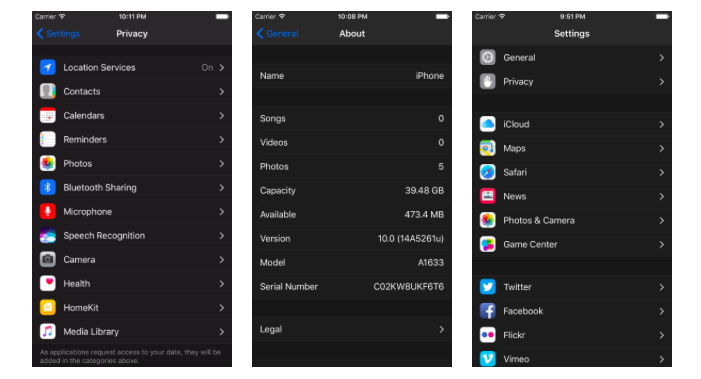This image set consists of three detailed screenshots taken from a person's cell phone, meticulously illustrating various settings menus:

1. **Left Screenshot: Privacy Settings Menu** - The first screenshot prominently displays the "Settings" menu focused on "Privacy." Listed under this heading are various subcategories including "Location Services," "Contacts," "Calendars," "Reminders," "Photos," "Bluetooth Sharing," "Microphone," "Speech Recognition," "Camera," "Health," "HomeKit," and "Media Library." It also includes a footer note stating, "As applications request access to your data, they will be added in the categories above."

2. **Middle Screenshot: General Settings Menu** - The middle screenshot is titled "General" and provides an overview of the device information. It includes sections such as "About," "Name," with the device identified as "iPhone," along with detailed storage information: "Songs" (0), "Videos" (0), "Photos" (5). It specifies the storage capacity as "39.48 GB" with "473.4 MB" available. The software version "10.0" with build number "14A5261u," model number "A1633," and serial number "CO2KW8UKF6T6" are also displayed. Additionally, there is a "Legal" section at the bottom.

3. **Right Screenshot: General Settings Expanded Menu** - The third screenshot further elaborates on the "Settings" menu with the "General" category opened. Visible sub-categories include "Privacy," "iCloud," "Maps," "Safari," "News," "Photos & Camera," "Game Center," "Twitter," "Facebook," "Flickr," and "Vimeo."

Each screenshot provides a clear view of the phone's configuration options, offering a comprehensive look at its privacy settings, device information, and additional general settings.